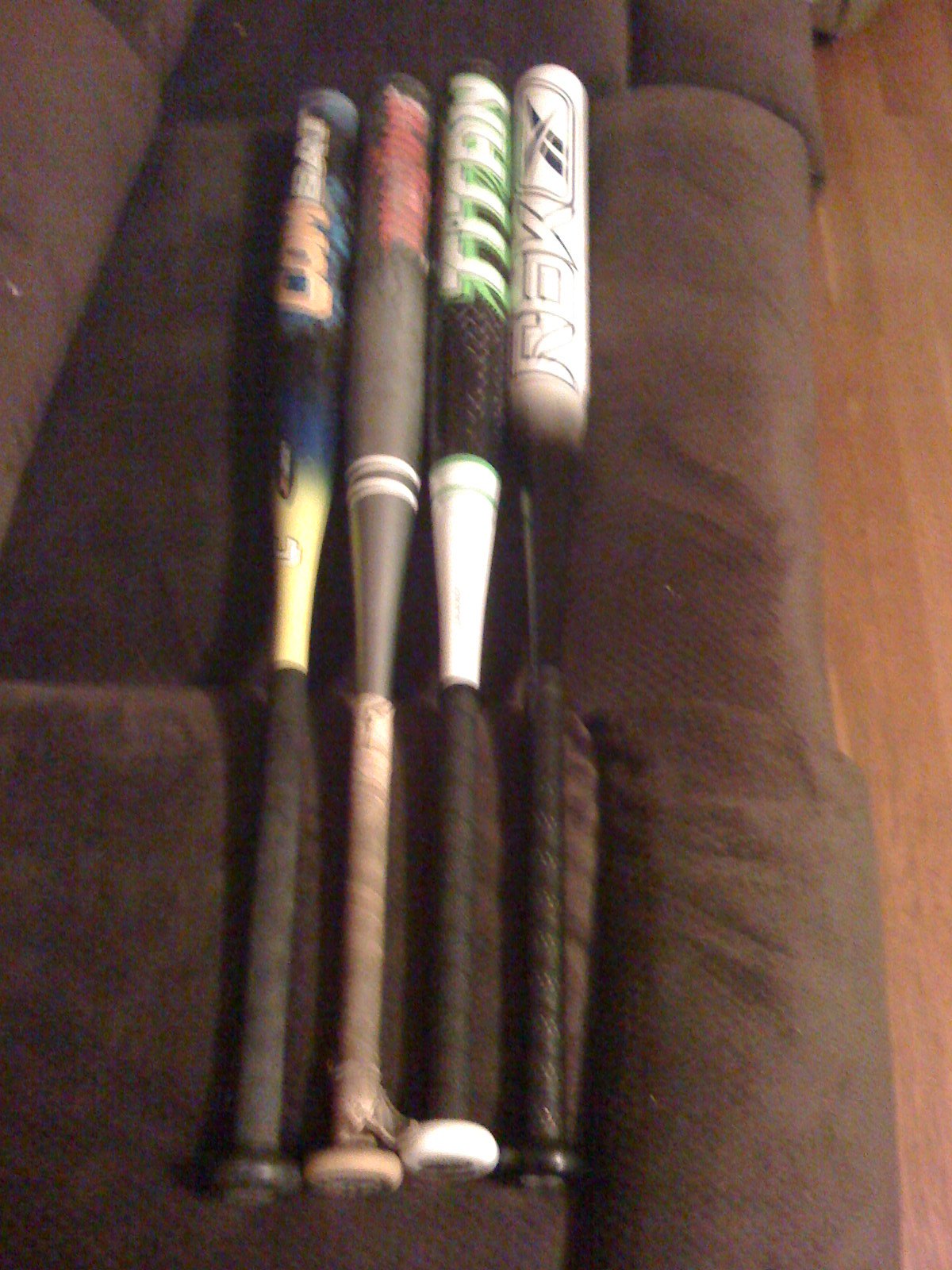The photo shows a slightly blurry, low-quality view looking down onto the seat of a dark brown sofa. Arranged side-by-side on the sofa are four distinct metal baseball bats. Each bat has unique characteristics and colors. The first bat, located all the way on the left, is mostly black with accents of blue and yellow, featuring the word "COMBAT" in yellowish-peach and white letters. The second bat is silver with a beige handle and red symbols at the top, although the text is not legible due to the photo's fuzziness. The third bat has a striking black and white design with green graffiti-like letters spelling out "TITAN," and it also features a black handle. The final bat on the right is branded with the Reebok logo; it’s primarily white fading into black with the letters "RBK" and a black handle. The sofa is placed on a wooden floor, visible underneath, and there are no other objects in the frame. This photograph may have been taken to display the variety of bats, possibly for sale or collection purposes.